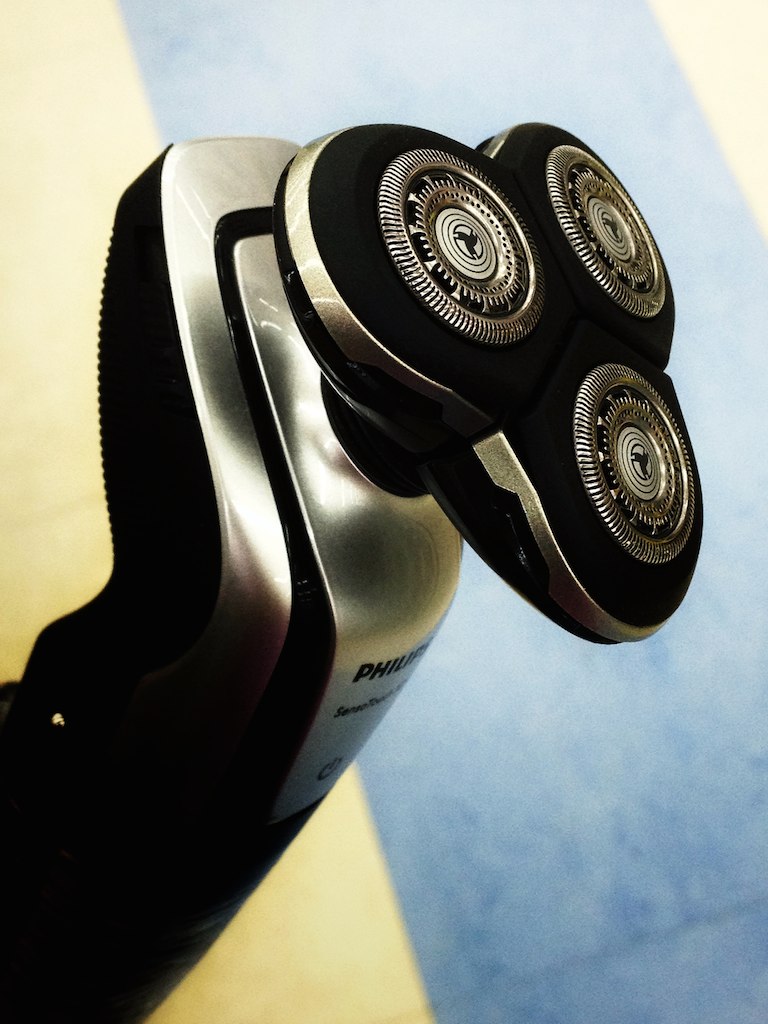This close-up image showcases an electric hair shaver against a blue and white striped background that is brightly illuminated. The shaver, prominently displayed in the center, features three circular shaving heads, each with a silvery metal surface adorned with intricate small black vertical lines. These heads are encased in a black circular shape, which merges into the silver and black handle. The top portion of the handle is shiny silver steel, tapering into a black base. The brand name "Philips" is clearly visible in black text just below the shaving heads. Light reflects off the metallic surfaces, emphasizing the sleek and efficient design of this well-crafted grooming tool.